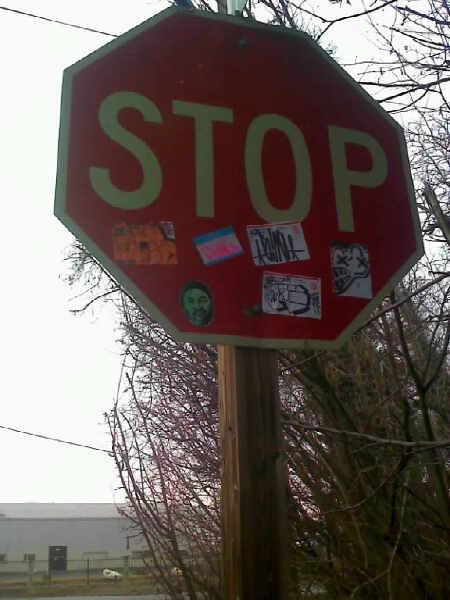This outdoor photograph captures an aged stop sign, taken from a low angle, mounted on a wooden post. The sign, featuring the classic red background and white lettering, is adorned with six various stickers beneath the word "STOP." These stickers, though not entirely clear, include depictions such as a face, scribbles, and colorful shapes. In the backdrop, the sky is overcast with gray tones, hinting at an overcast day. Surrounding the sign are bare trees or bushes, possibly indicating a fall or early spring season. Further in the background, a low, gray building and a fenced area with some indistinct animals suggest a rural or farm setting. Telephone wires also cut across the scene, adding to the rustic atmosphere.